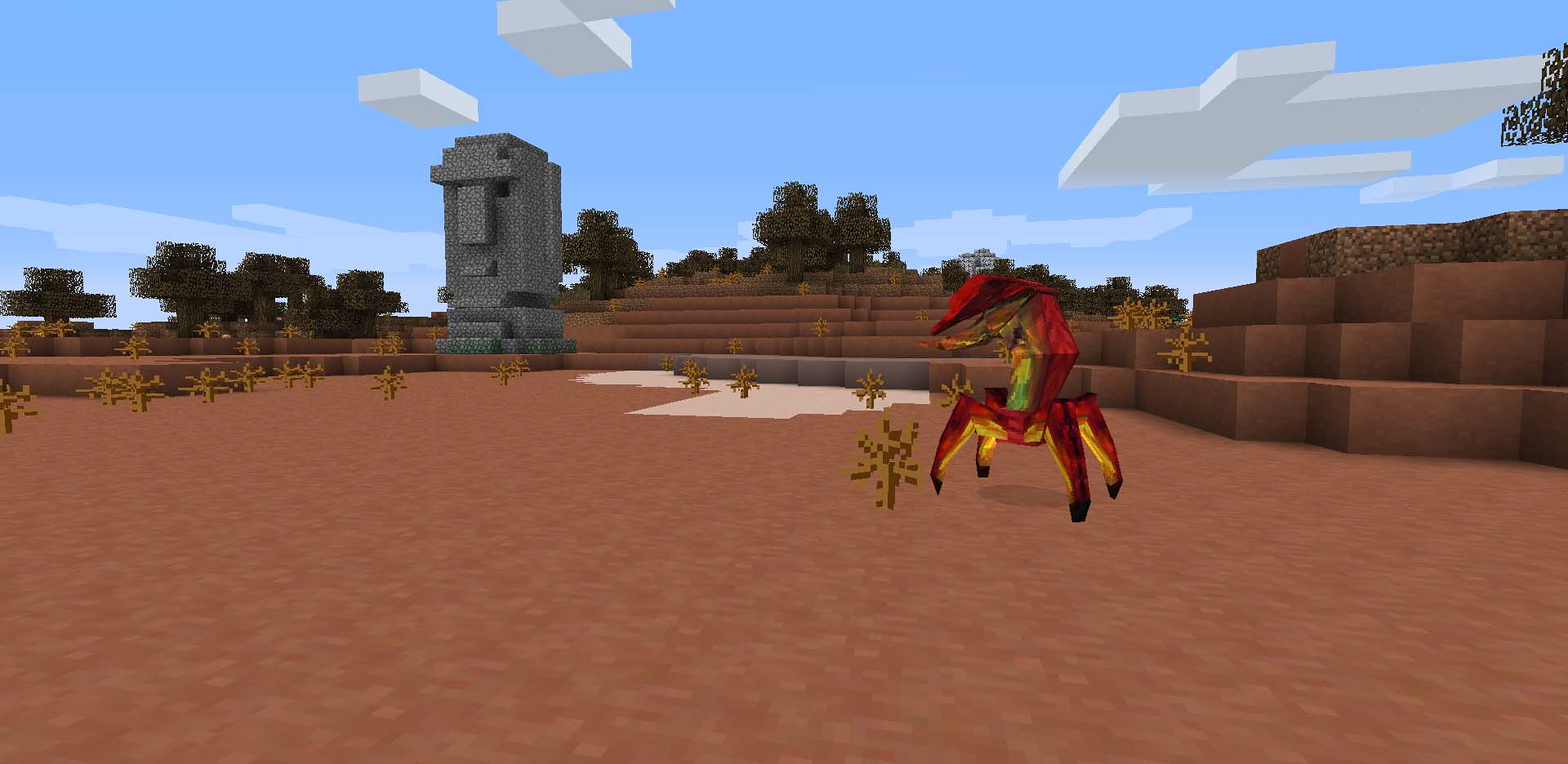In this detailed screenshot from Minecraft, an expansive brown terrain extends across the foreground, characterized by its geometric, blocky nature. Dominating the scene towards the center-right is a four-legged, red creature with a long neck, resembling a scorpion in its stance. Adjacent to this creature stands a small, green plant or flower, emblematic of the sparse vegetation scattered throughout this sandy area. Several similar small plants punctuate the barren landscape.

In the distant background, a white patch suggests either a snowy region or perhaps a different variety of sand, providing a stark contrast to the brown ground. Beyond this, a stone sculpture reminiscent of the iconic Easter Island statues with a blocky face stands prominently. Further along the horizon, a dense line of blocky trees marks the edge of the landscape.

The terrain here steps upward gradually, creating a tiered effect with the flat area where the creature stands at the base and successive levels rising behind it. At the very top of the frame, a bright blue sky filled with blocky white clouds completes the image, adding to the typical Minecraft aesthetic.